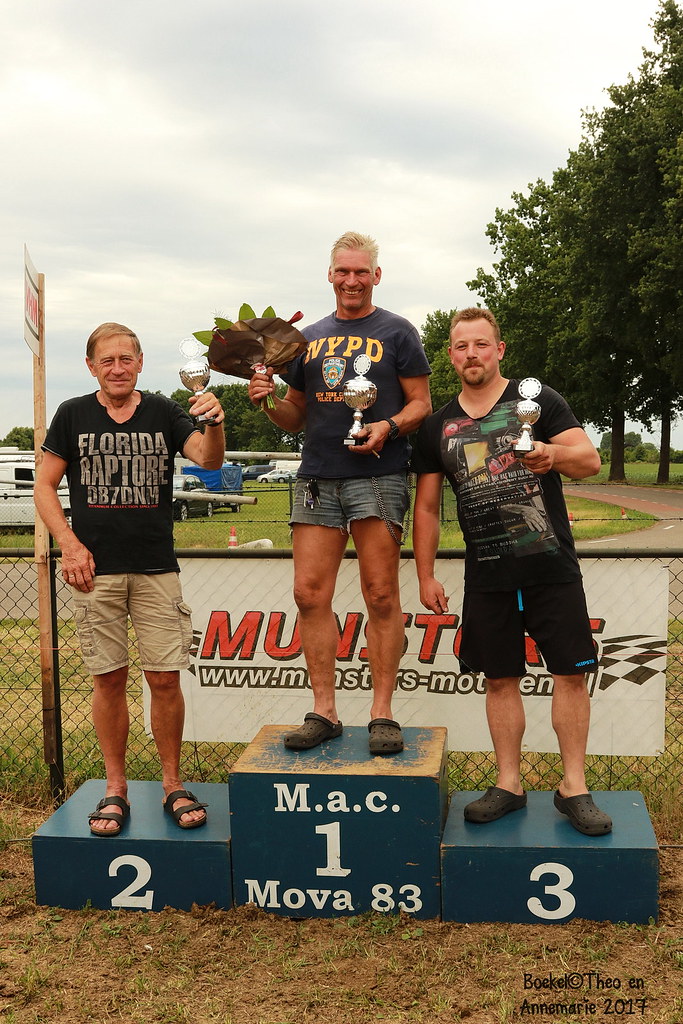In this image, three men stand on a winner's trophy podium, indicating their places in a competition. The podium consists of three blue boxes with white writing, with the tallest one in the center marked with "1" and "MAC MOVA 83." The man in the center, presumably the first-place winner, is middle-aged with bleached blonde hair, tanned skin, and wearing a tight blue NYPD t-shirt and denim shorts with a chain. He holds a silver trophy in his left hand and a bouquet of flowers in his right. To his left (our right), the second-place winner stands on a box labeled "2." He sports a longer black shirt that reads "Florida Raptor, DB7DNM," tan cargo shorts, and sandals. This man also has bleached blonde hair and holds a smaller trophy in his left hand. The third-place winner, positioned to the first-place winner's right (our left), stands on a box marked "3." He has a goatee, short-cropped dirty blonde hair, and wears all black: a t-shirt with text, shorts, and Crocs. He is smiling and holding a trophy identical to the second-place winner's. The background reveals a cloudy sky, a few trees, vehicles, and a track, suggesting a racing event. Behind them is a chain-link fence with a white sign featuring a black and white checkered flag, a website, and red writing, likely indicating a raceway or racing competition.